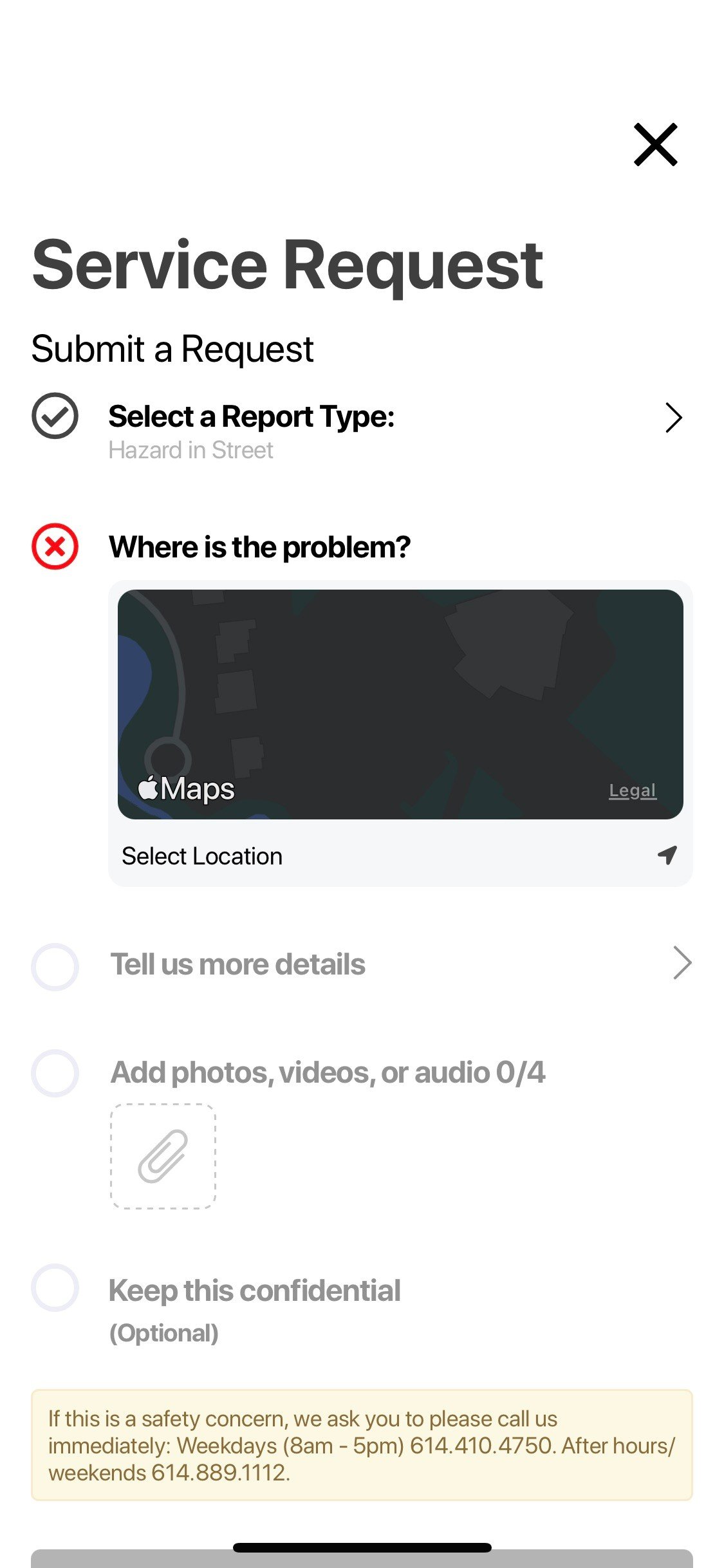The image appears to be a screenshot from a mobile device, likely a smartphone or tablet, given the aspect ratio and the presence of a navigation bar typically found on such devices. The interface is predominantly white, with black or gray text and minimal color, restricted mostly to icons and highlights.

At the top of the screen is the heading "Service Request," with a black 'X' in the upper right corner, indicating the option to close the dialog box. Below the heading, the text "Submit a Request" is displayed, followed by a field labeled "Select a Report Type" with a checkmark next to it. The chosen report type is displayed as "Hazard and Street."

Following this is a section titled "Where's the Problem?" accompanied by a red 'X'. Underneath, there is an embedded map interface, likely from Google Maps or Apple Maps, featuring buttons labeled "Legal" and "Select Location."

Further down, there is a text bubble inviting users to "Tell Us More Details," with options to "Add Photos, Videos, or Audio" (indicated as "0 out of 4"). There is also a checkbox labeled "Keep This Confidential."

Towards the bottom, a yellow highlighted section provides a cautionary note: "If this is a safety concern, we ask you to please call us immediately weekdays 8 a.m. to 5 p.m. 614-410-4750. After hours last weekend 614-889-112."

This image seems to depict a service request form within an app, illustrating the various fields and options available for users to report issues.